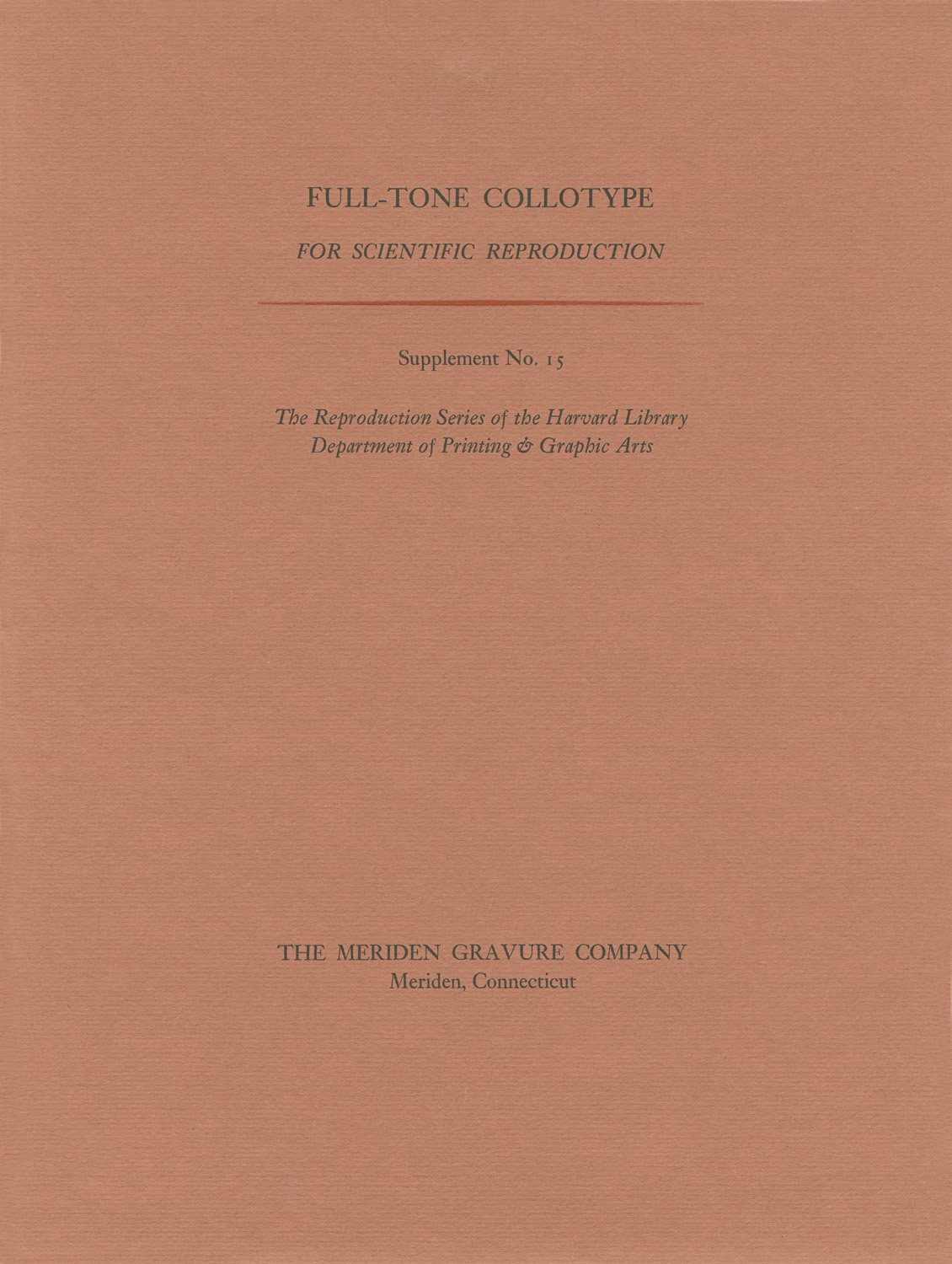The image is a photograph of a simple, front-facing book cover with a dark tan, leathery texture. At the top of the cover, the text reads "Full-Tone Collotype for Scientific Reproduction." A large red line divides this title from the subtitle "Supplement Number 11." Below this, the text states, "The Reproduction Series of the Harvard Library Department of Printing and Graphic Arts," and at the bottom of the cover, the publisher is listed as "The Meridian Gravure Company, Meridian, Connecticut." The overall design is minimalistic with a focus on the text, characterized by its uniform dark tan color and lack of illustrations, hinting at a scholarly or scientific publication.